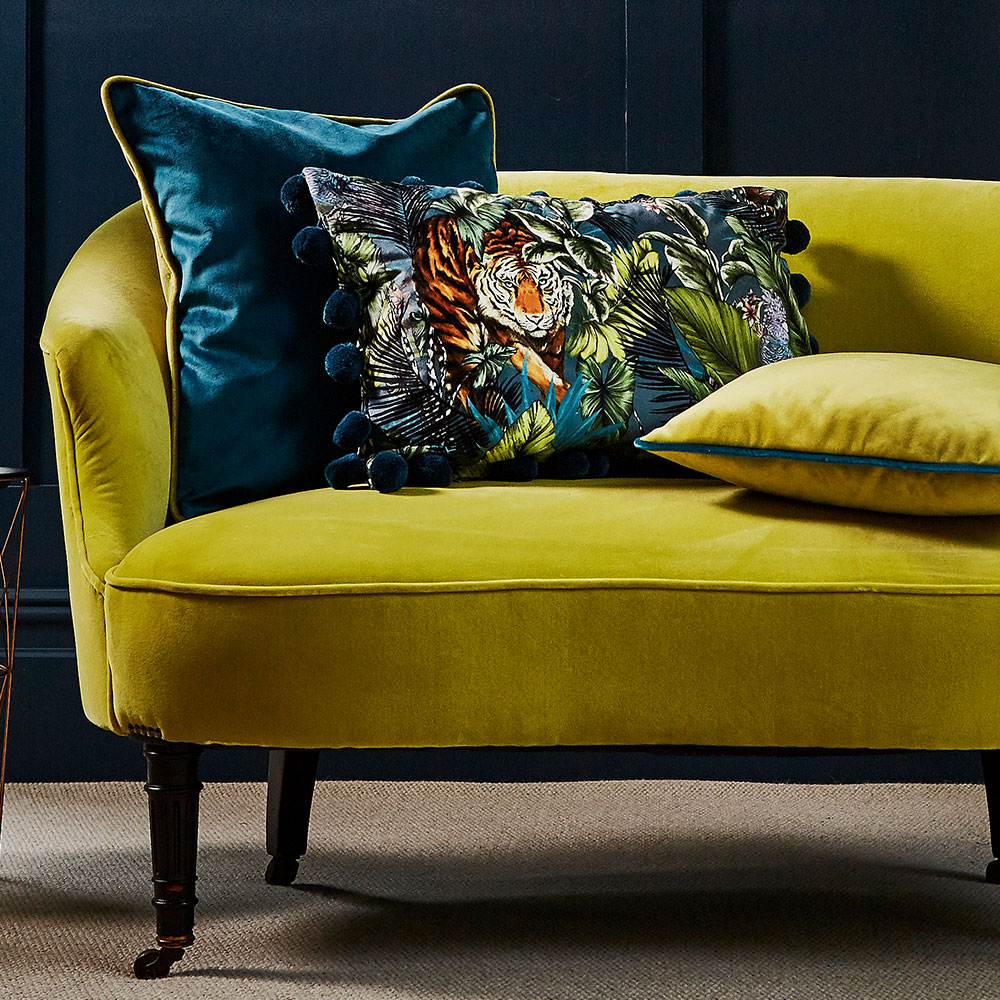This centered square photograph captures a partial view of a vintage-style sofa nestled in a room. The sofa, predominantly visible, showcases a left-side curvature and is upholstered in a non-tufted microfiber fabric of a greenish-yellow to olive shade, leaning towards mustard. It stands on dark wooden legs fitted with small rolling wheels, elevating its old-school charm. 

The sofa is set against a wooden wall painted in a deep navy blue, providing a striking backdrop. The couch is adorned with three distinct pillows: one matches the sofa's fabric with a teal trim, another reverses the colors with a blue fabric and greenish-yellow piping, and the middle pillow features a tiger prowling through a forest, accented with blue pom-poms.

Beneath the sofa lies a simple scrunched-up gray carpet, though some descriptions hint at a beige or low-pile brown variation. There's a side table partially visible to the side, described variably as possibly metal with a black top, adding to the eclectic decor. Shadows from the sofa add depth to the scene, underlining its prominence in the room.